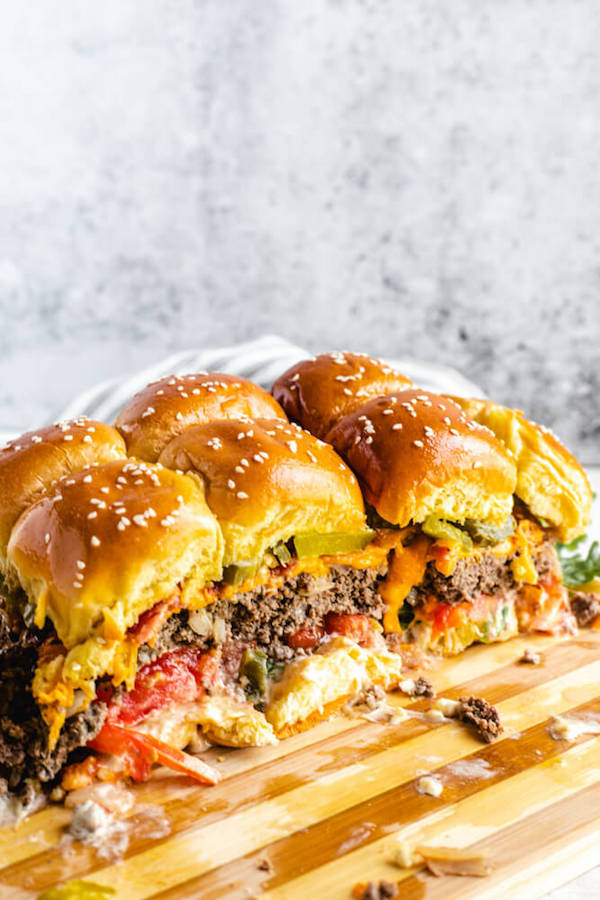The photograph showcases an appetizing array of six hamburger sliders, neatly arranged on a striped wooden cutting board. The sliders feature golden-brown sesame seed brioche buns, which have been cut or bitten into, revealing an enticing view of the contents within. Inside each slider, you can see layers of melted cheese, juicy ground beef patties, pickles, tomatoes, and a hint of tomato sauce just above the bottom bun. These substantial sliders, each with its own bun, appear large and hearty, suggesting they could have once comprised a larger sandwich. The background is a blurred, possibly marble gray or white wall that accentuates and brings focus to the vibrantly colorful burgers at the center. The photo has a clean, cookbook-like presentation, ideal for enticing any viewer to take a closer look or try the recipe themselves.